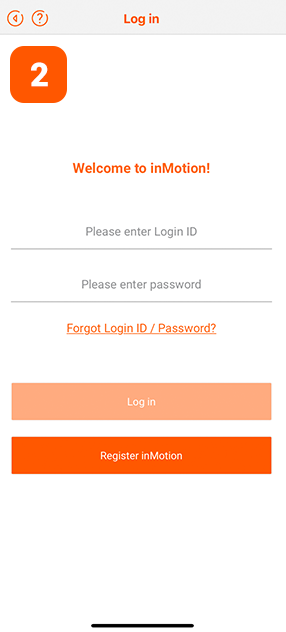The image showcases a login page for a website. At the very top, there is a horizontal gray bar spanning the entire width of the page. Within this bar, the word "Login" is displayed in orange letters. To the upper left, there are two orange circles: one with a left-pointing arrow and the other with a question mark.

Below this bar, a large, white number "2" is prominently displayed inside an orange square with rounded edges. Beneath the square, the text "Welcome to InMotion!" appears, with an exclamation point oriented vertically to the side. 

Following the welcome message, the prompt "Please enter login ID" is written in gray text, accompanied by a gray line below it for users to input their ID. Similarly, the prompt "Please enter password" is shown with a gray line underneath it for password entry.

Further down, the text "Forgot login ID/password?" appears, offering a clickable link that helps users retrieve their login information. 

At the bottom of the page, there is a light orange bar with the word "Login" in it, followed by a darker, orangey-red bar that says "Register InMotion." Clicking this bar allows new users to register and start using the service. A black line runs along the very bottom of the image, grounding the layout.